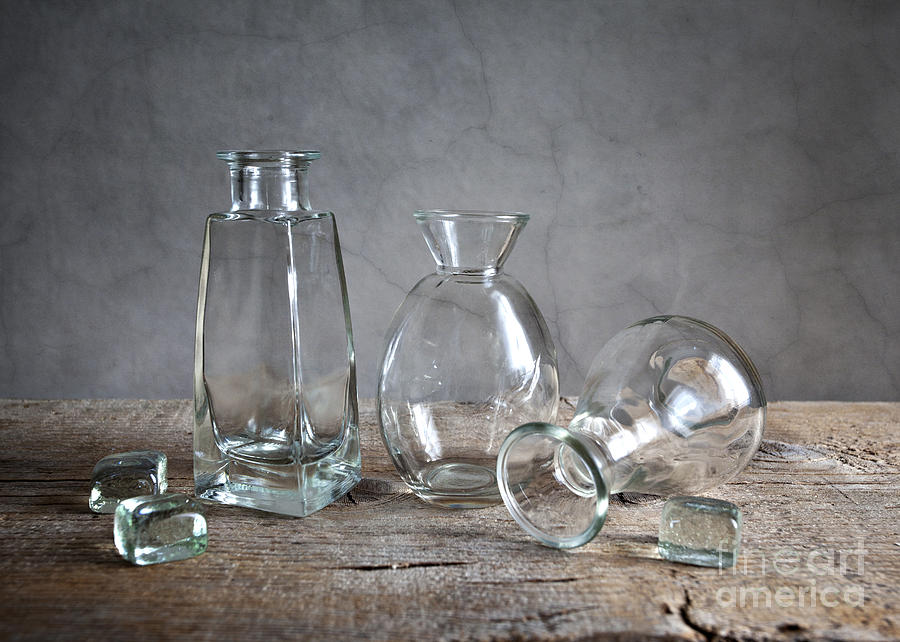The photograph captures three distinctive glass vases arranged on a rough wooden table, set against a multicolored gray stone wall with linear patterns. The leftmost vase, the tallest, has a narrow, rectangular shape with a flat cylindrical top. The center vase, egg-shaped, features a funnel-like descending top. The rightmost vase, teardrop-shaped, lies on its side and also has a funnel-shaped top. Surrounding the vases are three small, clear glass cubes—two situated to the far left of the arrangement and one on the right near the teardrop-shaped vase. A semi-transparent white watermark reading "fine art" and "america," both in lowercase, appears in the bottom right corner of the image. Despite their differences, none of the vases are particularly tall. The entire arrangement is placed on a stone-like counter, contributing to the rustic ambiance of the scene.